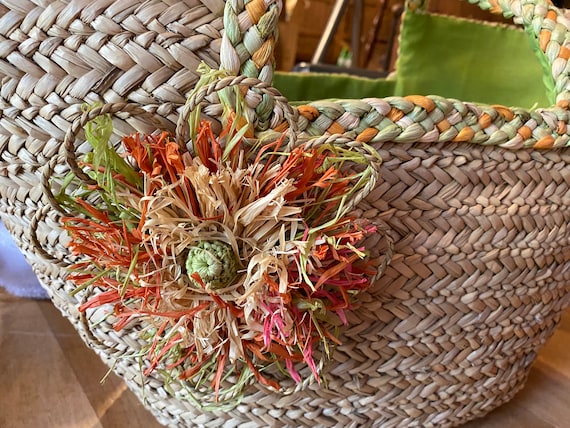This close-up image captures a woven basket, intricately handmade with a soft textile material arranged in a herringbone pattern. The light brown to grayish woven surface of the basket is complemented by a unique handle, accentuated with pastel accents of yellow, green, and gray. The focal point, however, is a large decorative flower that adorns the basket. This flower features a green knotted center made from the same textile, surrounded by braided hoops that imitate flower petals. These petals are fringed and frayed in a kaleidoscope of vibrant colors, including oranges, greens, yellows, and pinks, creating a wild yet purposefully colorful design. The basket rests on a wooden surface, with hints of green fabric lining peeking out, adding an additional element of texture and color to the scene.